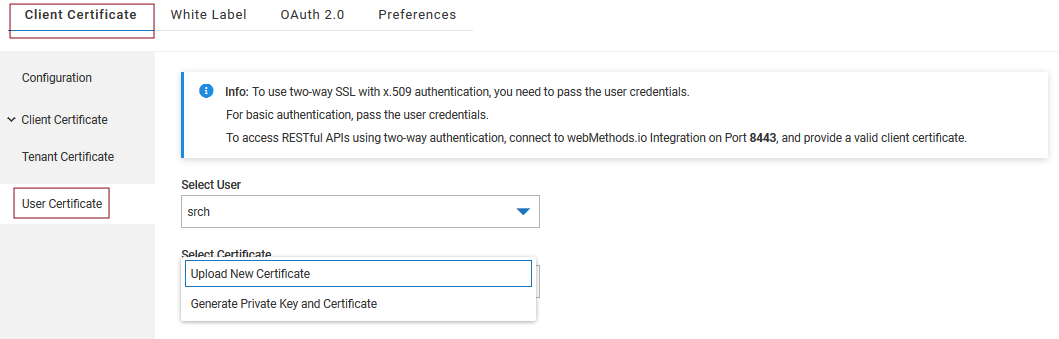**Detailed Caption:**

The image is a screenshot from a computer interface, presumably from a website or application related to certificates and authentication settings, featuring a white background at the top. At the top, the text "Client Certificate" is prominently displayed with capitalized 'C's. Below it, a thin blue line underscores this title, encased within a faded mauve or burgundy rectangle that highlights the section.

Underneath, several options are listed: "White Label," "OAuth 2.0," and "Preferences." On the left side of the interface, a light gray sidebar features various menu items. At the top of this sidebar, it says "Configuration" with a down arrow next to it, indicating a dropdown menu. Below that, "Tenant Certificate" is listed.

Another section featuring the same faded burgundy rectangle has "User Certificate" written inside it. Below this rectangle, there is an empty gray box. Adjacent to this, a white panel with a blue left-side border and a circular 'info' icon explains the usage conditions for Two-Way SSL with X.509 authorization or authentication. The panel outlines the need to pass user credentials for basic authentication and to connect to webmethods.io integration on port 8443 with a valid client certificate for accessing RESTful APIs using Two-Way authentication.

Further down, options such as "Select User," with a search field labeled "SRCH," are provided. Additionally, there are options to "Select Certificate," "Upload New Certificate" (marked with a blue line border), and "Generate Private Key and Certificate."